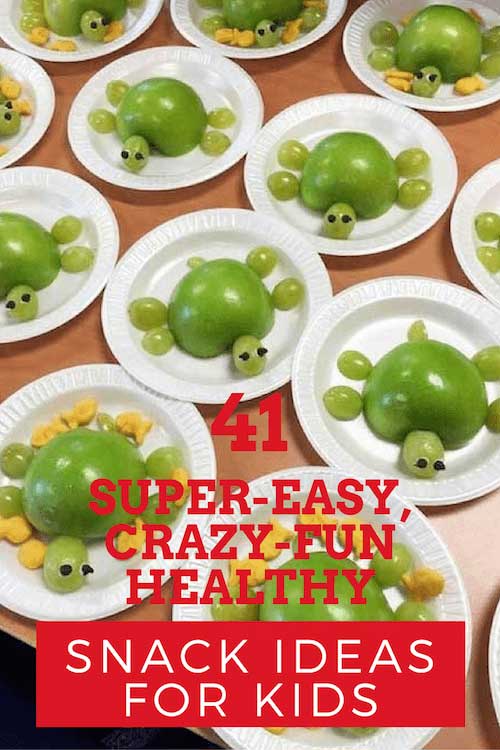This image features a vibrant and playful advertisement for a kids’ snack ideas book, blog, or magazine. The text overlay in red and white announces "41 Super Easy, Crazy Fun, Healthy Snack Ideas for Kids," with "Snack Ideas for Kids" prominently displayed in a red box with white letters, all in capital letters. The image itself showcases a table adorned with numerous white plates, each creatively arranged to resemble turtles. The body of each turtle is made from a half green apple, turned cut-side down, with four green grapes positioned around it as legs. The turtles' heads are crafted from a single grape, adorned with tiny black dots for eyes, possibly made from chocolate chips or another small edible item. Additional plates feature colorful corn pops or goldfish crackers, enhancing the fun and nutritious appearance aimed at appealing to kids and parents alike.